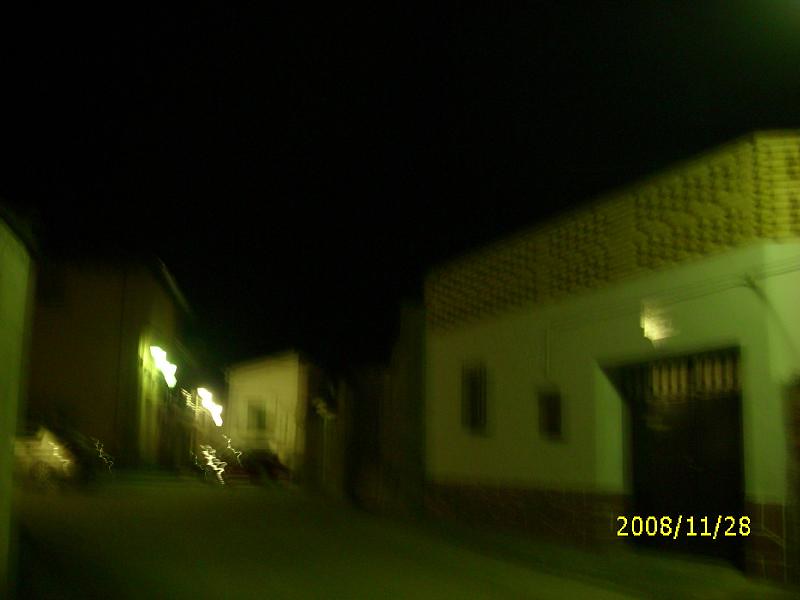This blurry, nighttime photograph captures a small street or alleyway. The sky is very dark, suggesting it was taken either late at night or early in the morning. A yellow timestamp in the lower right corner of the image reads "2008-11-28." Four buildings can be seen along the street, characterized by their flat tops, which give them an unusual architectural appearance that suggests the location might be outside the U.S. 

Closest to the camera on the left side, there is a silvery car parked in front of a white building with a brown base and a garage door topped with window slats. This building has a small window and a larger window, alongside a light above the garage door. Further down the street, two out-of-focus cars, one grayish and one blackish, are faintly visible under the illumination of two bright lights from another building in the distance.

On the right side of the image is another conspicuous building, featuring a garage door with two small windows and possibly a railing for a deck above it, though details are obscure due to the darkness. In the background, a small, possibly red car is faintly seen parked further along the street. The overall fuzziness and motion blur of the photograph make it difficult to capture finer details, leaving many elements indistinct and giving the impression of a hastily taken snapshot.